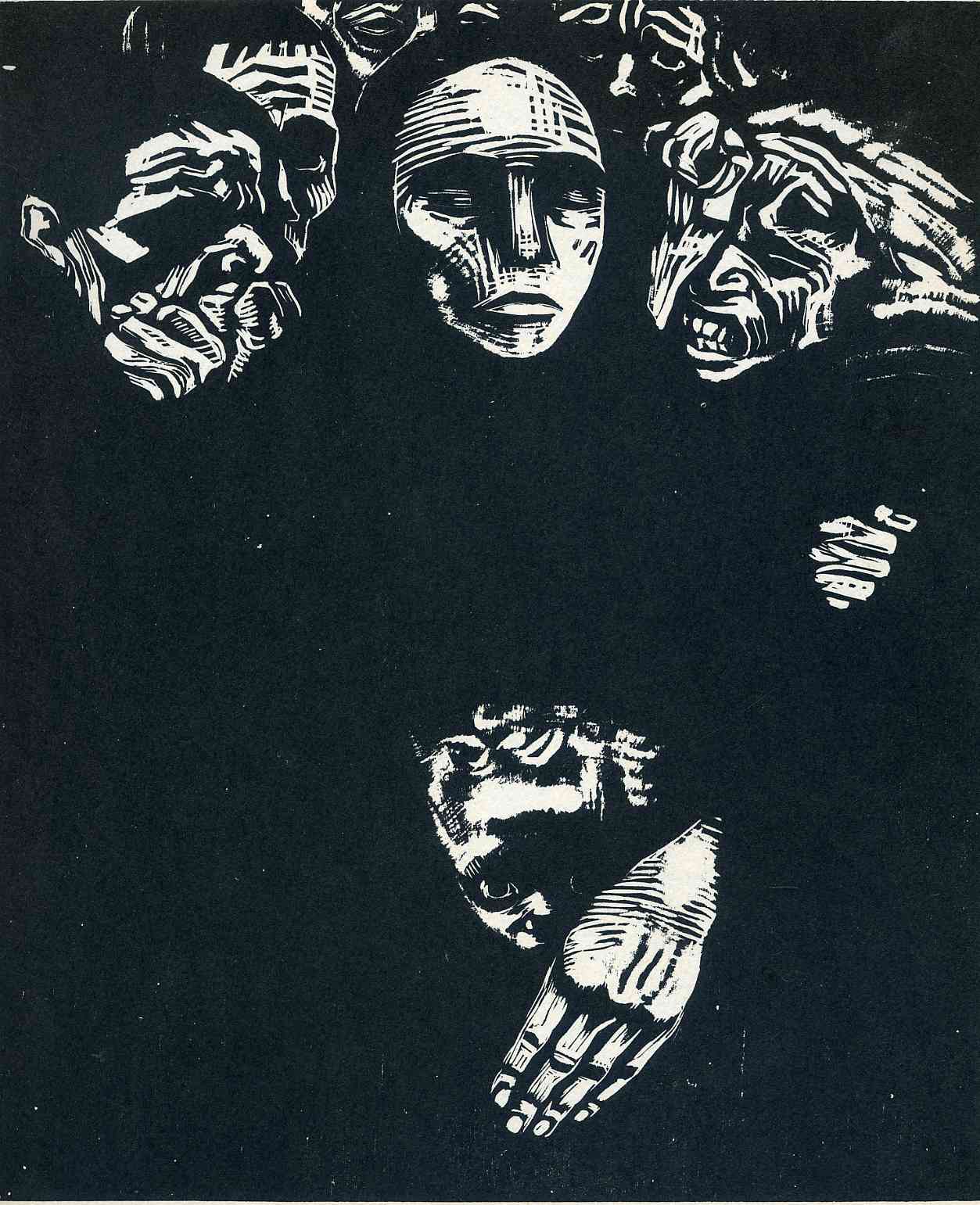The artwork is an intriguing piece with a predominantly black background, rendered in what appears to be a scratchboard technique, giving it a stark black-and-white contrast. At the top of the image, a series of faces emerge, each evoking different emotions—worry, anger, and contemplation—with some appearing almost grotesque or demonic. Particularly striking is a mask-like face in the center and a monstrous face with visible teeth and possible horns to the right. The eyes of these faces are largely obscured, adding to their eerie, abstract quality.

Moving downward, on the left side, two more faces appear, one with a noticeable deformity around the mouth, further enriching the haunting atmosphere. At the bottom center of the composition, a small, bright-eyed face of what seems to be a child is visible, starkly white against the black background. This child's face is partially covered by a large hand, which does not appear to belong to the child. This hand, potentially protective or menacing, extends from one of the larger faces above. The overall piece, with its minimalistic yet expressive detail, undoubtedly conveys a deeper, symbolic meaning open to interpretation.